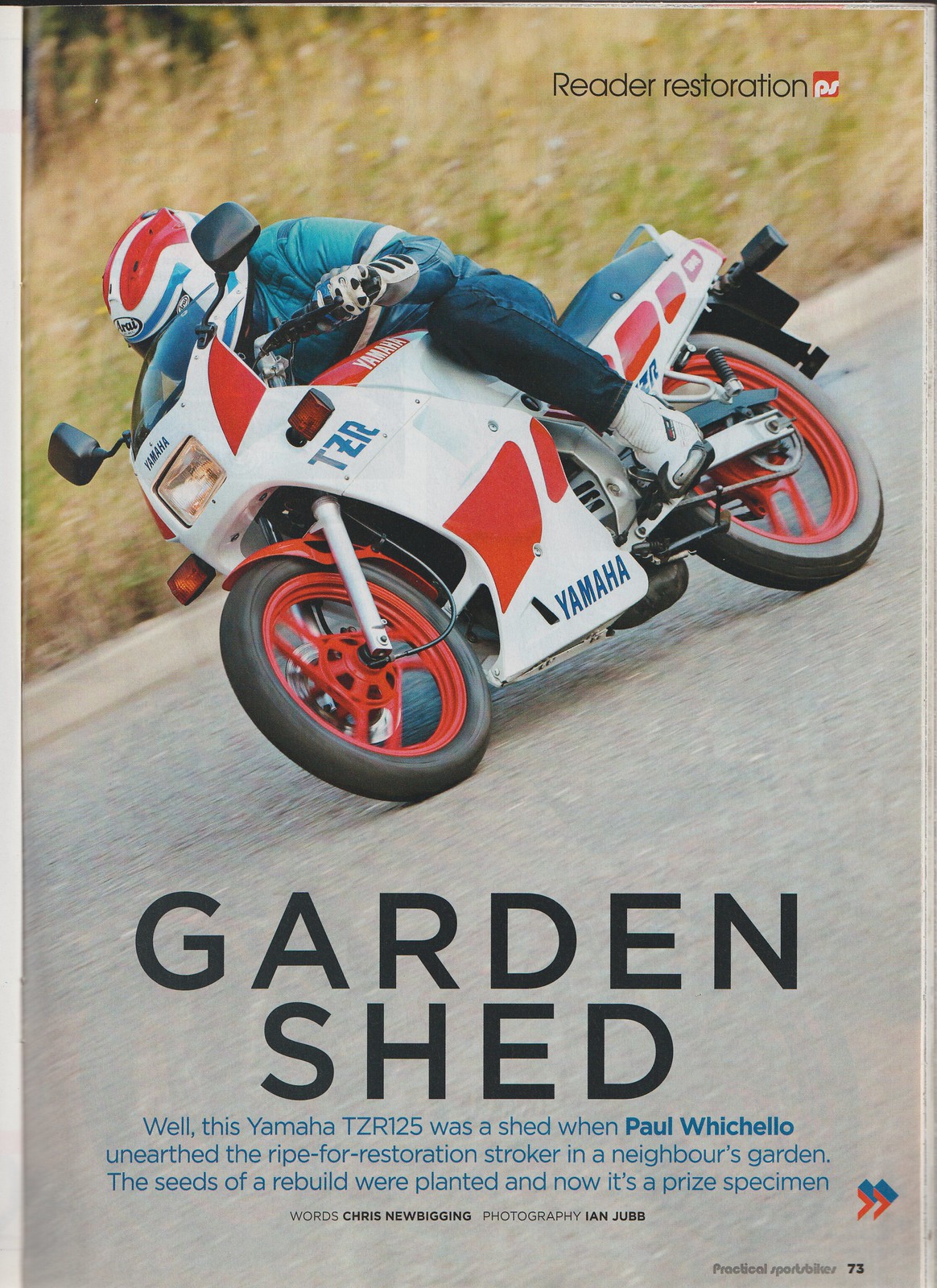In a scan of a retro-styled magazine advertisement, a man on a white and red Yamaha TZR125 motorcycle leans into a turn on a gray road, evoking a sense of high-speed motion against a backdrop of a grassy field. The rider, clad in a green puffy coat, blue jeans, white shoes, and a striking helmet with red, white, and blue stripes, is the image's focal point. On the top right, the text reads "Reader Restoration, PS," while the bold headline "Garden Shed" sits prominently below the cyclist. Accompanying the image, a caption recounts how Paul Wichelow discovered the motorcycle in a neighbor's garden, transformed it from a dilapidated state into a prized specimen. Words by Chris Newbigging and photography by Ian Jubb are credited in smaller text. Additionally, two red arrows with blue shadows appear subtly on the bottom right, and in shadowy gray text at the very bottom, it notes "Practical Sports Bikes" with a small "73," marking the publisher. The scan also reveals magazine staples on the left margin, emphasizing its vintage appeal.